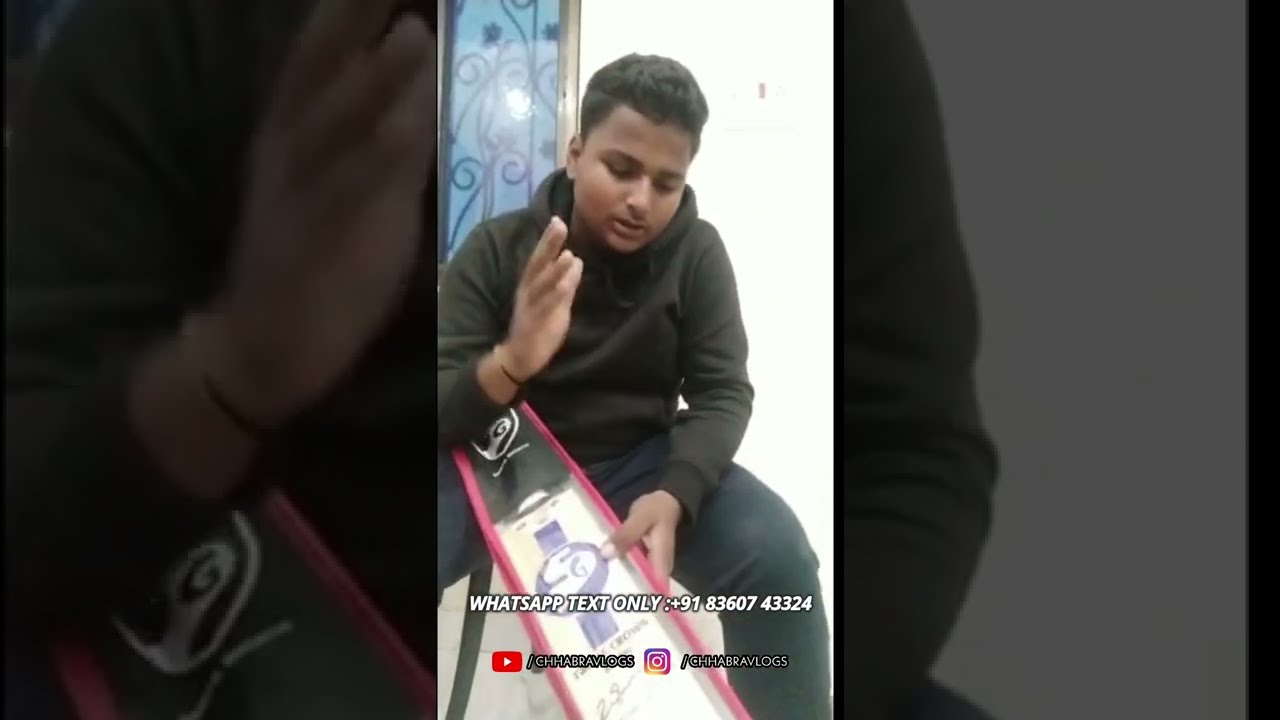A young man, possibly in his late teens or early 20s, with dark brown skin and black hair brushed upward, is sitting down and holding up a board in one hand. He is wearing a black hoodie and black pants, with a gold bracelet on the hand that is held up next to his cheek as if gesticulating or explaining something. His eyes are directed downwards towards the object in his hand. This object, which could be a skateboard or a ski, has a pink-bordered design with a lighter center color, adorned with a white 'S' surrounded by a purple circle and a black section featuring a white 'G'. In front of him, text on the image reads "WhatsApp text only: +918360743324". Below this text are the YouTube and Instagram symbols followed by his usernames. The background features a white wall, and to the left, there is a window with intricately designed metal barriers and a slight glare reflecting off the glass. The photo is horizontally rectangular.